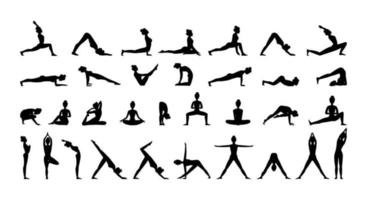This image is an infographic showcasing various yoga poses laid out in a landscape orientation against a solid white background with no defined border. The poses are depicted as black silhouettes, lacking detailed features but clearly illustrating each individual posture. The infographic is organized into four rows of stretching and yoga poses. 

The top two rows each contain seven poses, depicting a variety of common yoga postures like downward-facing dog and basic standing stretches. The third row has nine poses, while the bottom row features ten poses. The silhouettes vary between head-on and profile views, demonstrating a range of movements such as standing, bending over, lunging, and raising arms in different directions. There is no text or color aside from the black and white, making the focus solely on the visual representation of the yoga poses, suitable for a yoga studio or instructional webpage.